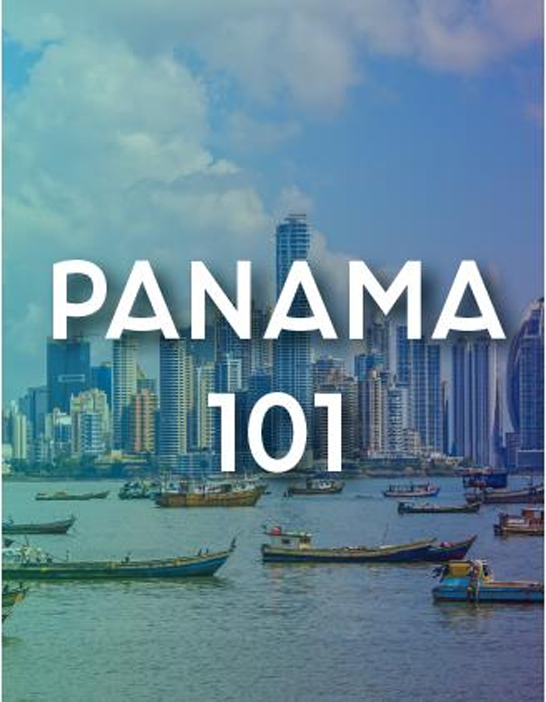A mesmerizing digital poster or wallpaper showcasing a serene city skyline by the sea, with the text "PANAMA 101" in bold, uppercase white letters adorned with a subtle gray drop shadow. The photograph reveals a modern, bustling city, featuring a plethora of towering skyscrapers. Several of these high-rises are accompanied by cranes, hinting at ongoing renovations or construction. Below the impressive skyline, the tranquil sea is dotted with various boats, ranging from small fishing vessels to elongated passenger boats. The entire image is bathed in a unique bluish-green filter, giving it a distinct, ethereal quality. Fluffy clouds adorn the sky, completing this captivating urban seascape.